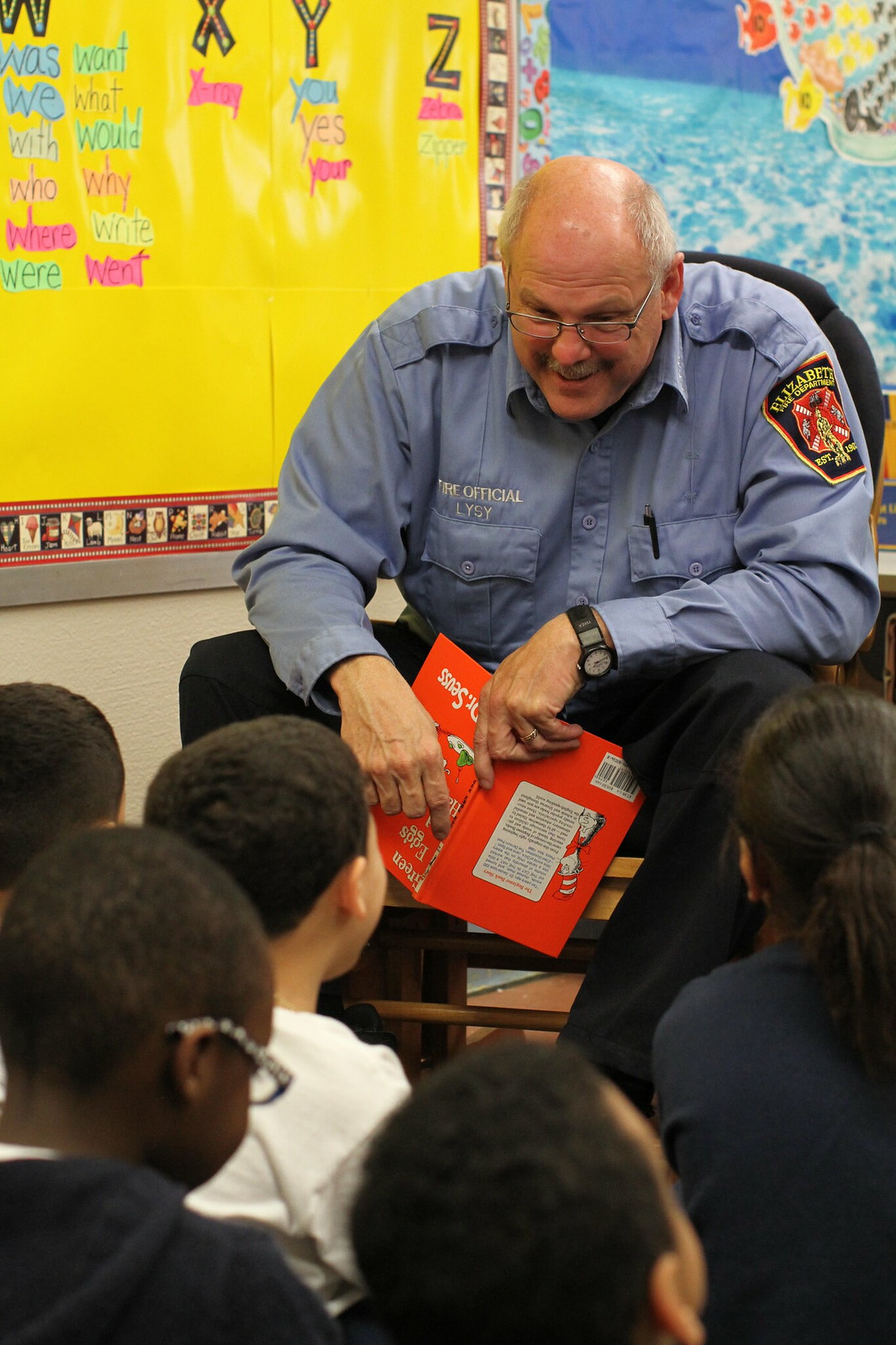In this heartwarming image, a bald, middle-aged fireman, donned in a blue long-sleeve shirt adorned with his name "L-Y-G-Y" and the fire department's emblem on his left bicep, is seated on a chair in a vibrant school classroom. He sports wire-rimmed glasses, a gold wedding band on his right hand, and a black wristwatch on his left wrist. The fireman is joyfully reading an open, red Dr. Seuss book, possibly "Horton Hears a Who," to a captivated group of schoolchildren. The children, seated on the floor around him, appear to be thoroughly engaged, paying close attention to the story. In the background, colorful classroom decorations, including a prominent yellow board with letters and words at different angles, various student projects, and a blue poster that resembles water in a pool, add to the cheerful and educational environment of the scene. The fireman's content expression and the children's rapt attention highlight the warmth and positive interaction taking place in this educational setting.